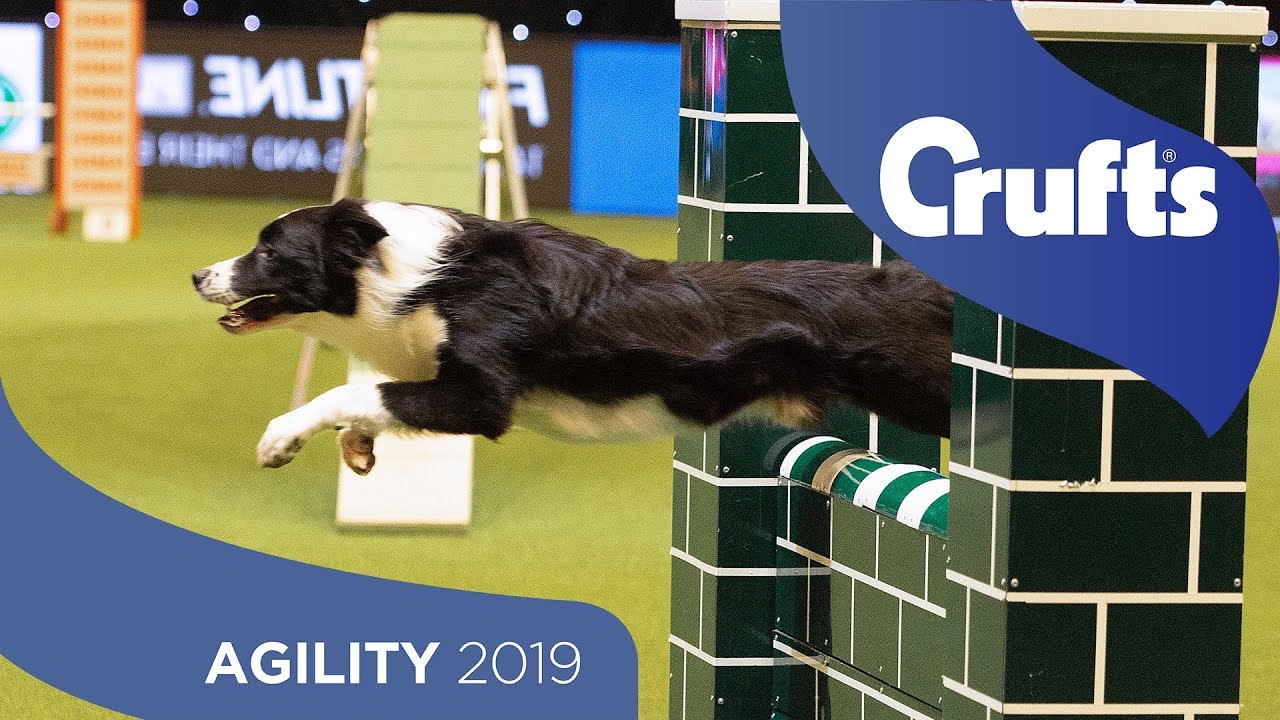The image captures an action shot from an indoor dog show, prominently featuring a black and white dog, possibly a shepherd or Labrador mix, in mid-leap through a meticulously designed obstacle. The dog is characterized by its black head and body, contrasted with a white nose, neck, underbelly, and paws. The obstacle consists of black brick-like columns with white borders and a lower section adorned with a green and white flag. The background reveals a greenish-yellow floor and several other structures, such as steps and slides, indicating a well-equipped agility course. To the left, a yellow and orange banner with writing adds to the competitive atmosphere. At the top, a blue banner with "Crufts" in bold white letters signifies the event, while a similar banner at the bottom right reads "Agility 2019," underscoring the year and nature of the competition.